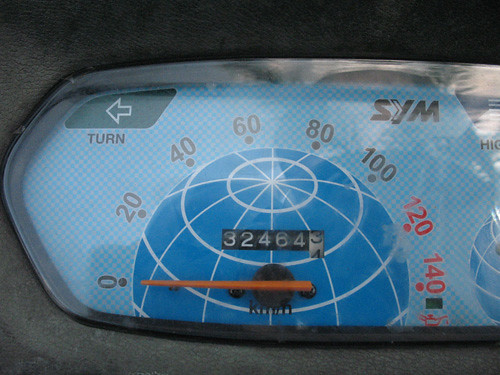The image captures the left side of a car's gauge cluster with intricate details. The base of the cluster features a dark border with a subtle green hue. Above this, is a glass-covered gauge area. Dominating the gauge area is a speedometer with a distinctive globe shape at its center. The globe is a striking blue, interlaced with white lines, and is marked with speed increments ranging from 0 to 140. In the center of the gauge, an odometer displays the number sequence 3, 2, 4, 6, 4, with the white roller positioned between the digits 3 and 4. On the top left is a turn signal indicator marked by the word "TURN" below an arrow that appears to illuminate. The background within the gauge cluster showcases a blue, angled checkerboard pattern, adding depth and texture. On the top right, the letters "SYM" are prominently displayed, just beneath the upper border, which matches the color of the lower border.